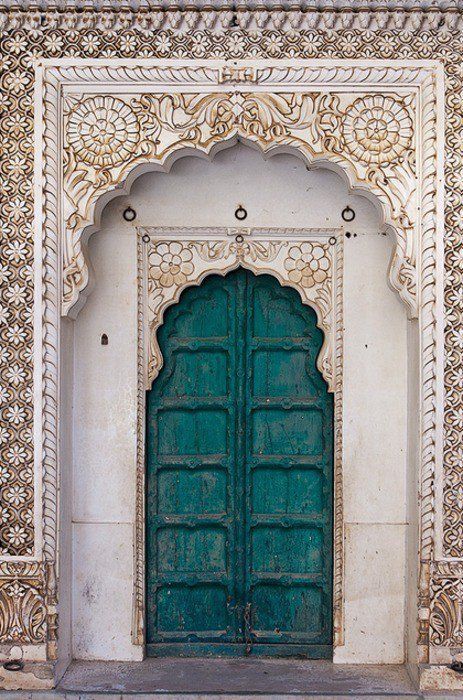The photograph captures an ornate, double-panel door set within a deeply recessed doorway. The door itself is a dark teal-green, reminiscent of patina brass or faded iron, and features intricate panel designs, possibly numbering around twelve. The door is slightly ajar and appears to swing open from the center. Below, a small section of chain lies draped across the bottom.

Framing this visually striking door is a detailed, arched door frame richly decorated with floral and scrollwork engravings that evoke the aesthetics of both Catholic cathedrals and Islamic architecture. The predominant colors of this lavish frame are white and cream, with subtle gold and gray shadowing that accentuates the depth and intricacy of the designs. Above and on either side of the doorway, large metal rings suggest functional elements, likely used in the past to secure the door with chains.

The wall surrounding the door is similarly elaborate, displaying a continuation of the flowery, marble-like engravings that give the entrance a historical and almost mystical quality. At the base of the doorway, there is a cement walkway, emphasizing the door's placement within an indentation or offset from the main path, adding to the sense of depth and antiquity.